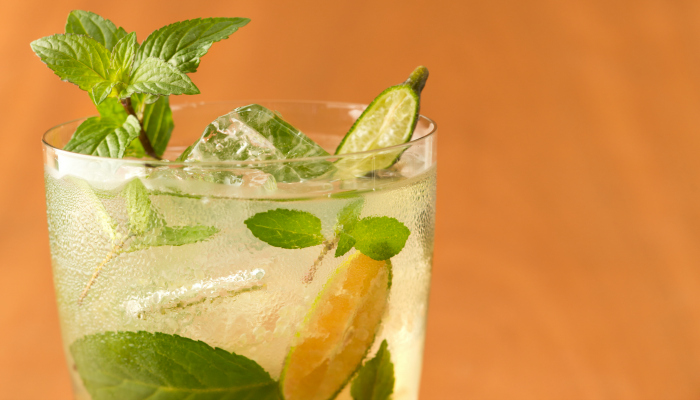The photograph showcases a high-definition, close-up view of a refreshing beverage in a clear, deckle-edged glass set against a vibrant orange, matte backdrop. The drink appears to be a summery cocktail, potentially a caipirinha or mojito, adding to its tantalizing appeal. The glass is filled almost to the brim with a bubbly liquid, suggesting a cold, perhaps seltzer-based drink. Inside, there are slices of lemon and lime, complemented by fresh, green mint leaves and possibly eucalyptus sprigs. A large ice cube floats at the top, enhancing its crisp and invigorating appearance. The entire scene exudes a vibrant, summery feel with its interplay of yellow, green, and orange hues – a visually inviting picture perfect for a Pinterest cocktail tutorial.